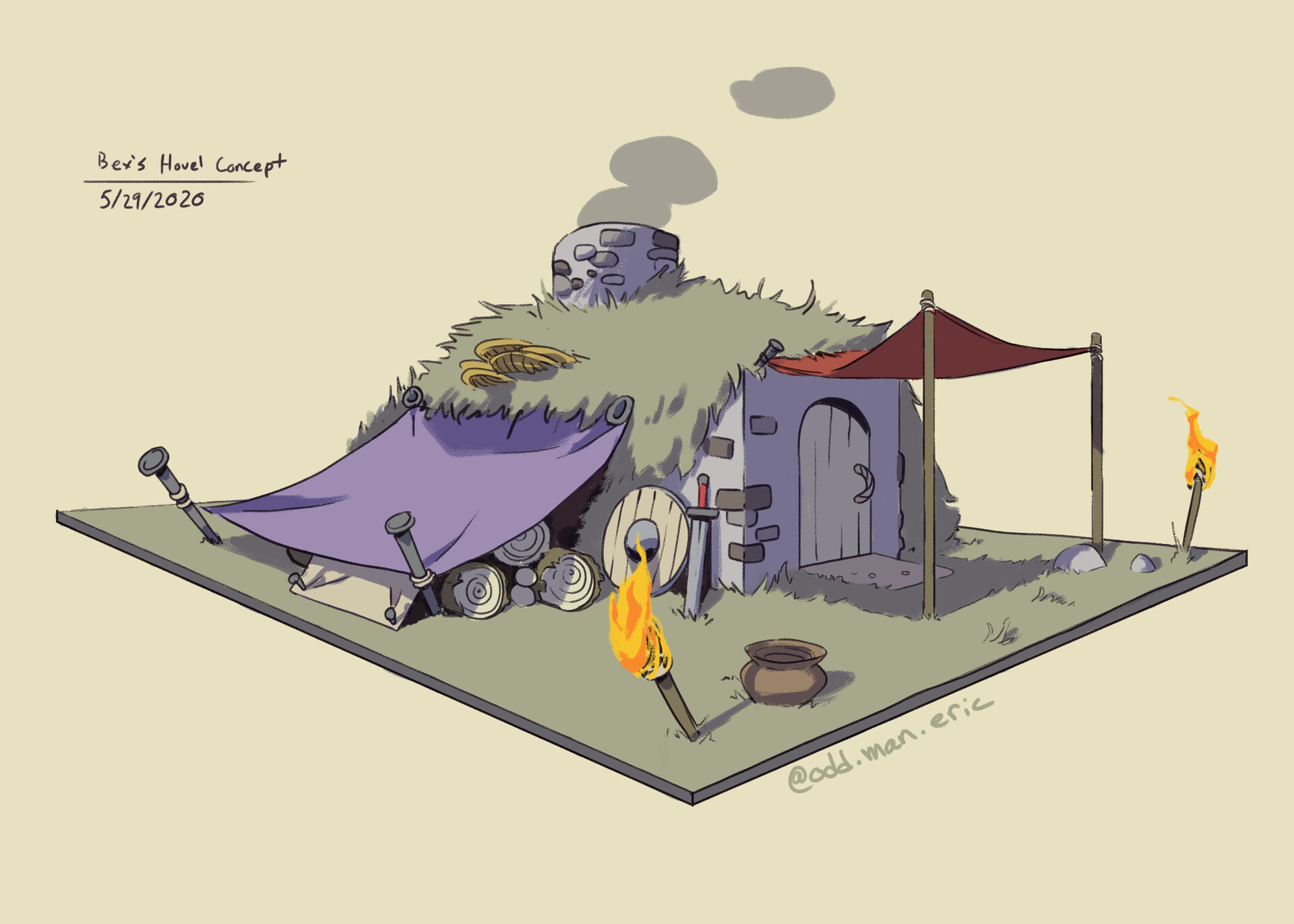The image is a detailed concept illustration labeled "Bex's Hovel Concept," dated 5-29-2020. This artwork, seemingly created during the early pandemic period, depicts a small, decrepit stone structure with a chimney, possibly serving as an RPG (role-playing game) element. The hovel features a single door, a purple tent with logs underneath, and a front canopy supported by two poles with a red top. Lit torches are positioned on both sides, casting a warm glow. A shield and a sword lean against the hovel's wall, suggesting a medieval or fantasy setting. Smoke emanates from the chimney, enhancing the rustic ambiance. The scene is presented in an axonometric view on a square piece of land, with a website watermark "at odd.man.eric" in the lower right corner. This quaint, color-faded illustration serves as a small but immersive depiction of a character's humble abode within a larger game-world environment.